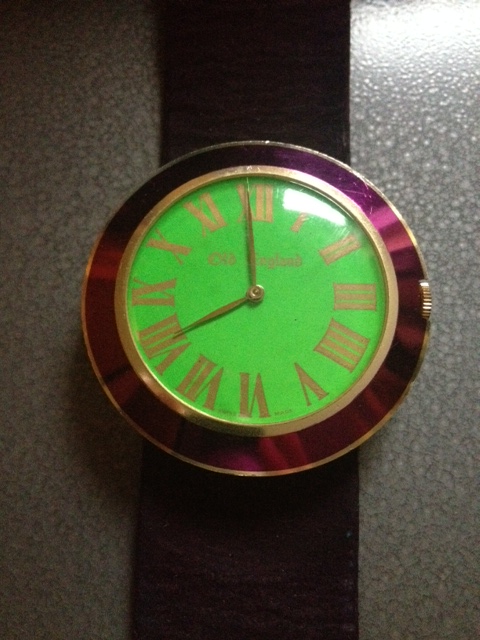Close-up photograph of a wristwatch with a black leather band, laid flat on a gray, shiny, textured surface that appears to be plastic. The watch face features a green background adorned with brass-colored Roman numerals and watch hands. Faint lettering is visible on the background, with "England" clearly discernible on the right side. Surrounding the dial is a metallic, rose-maroon textured border that resembles paneling. This is encircled by a thin, brass-colored metallic band.